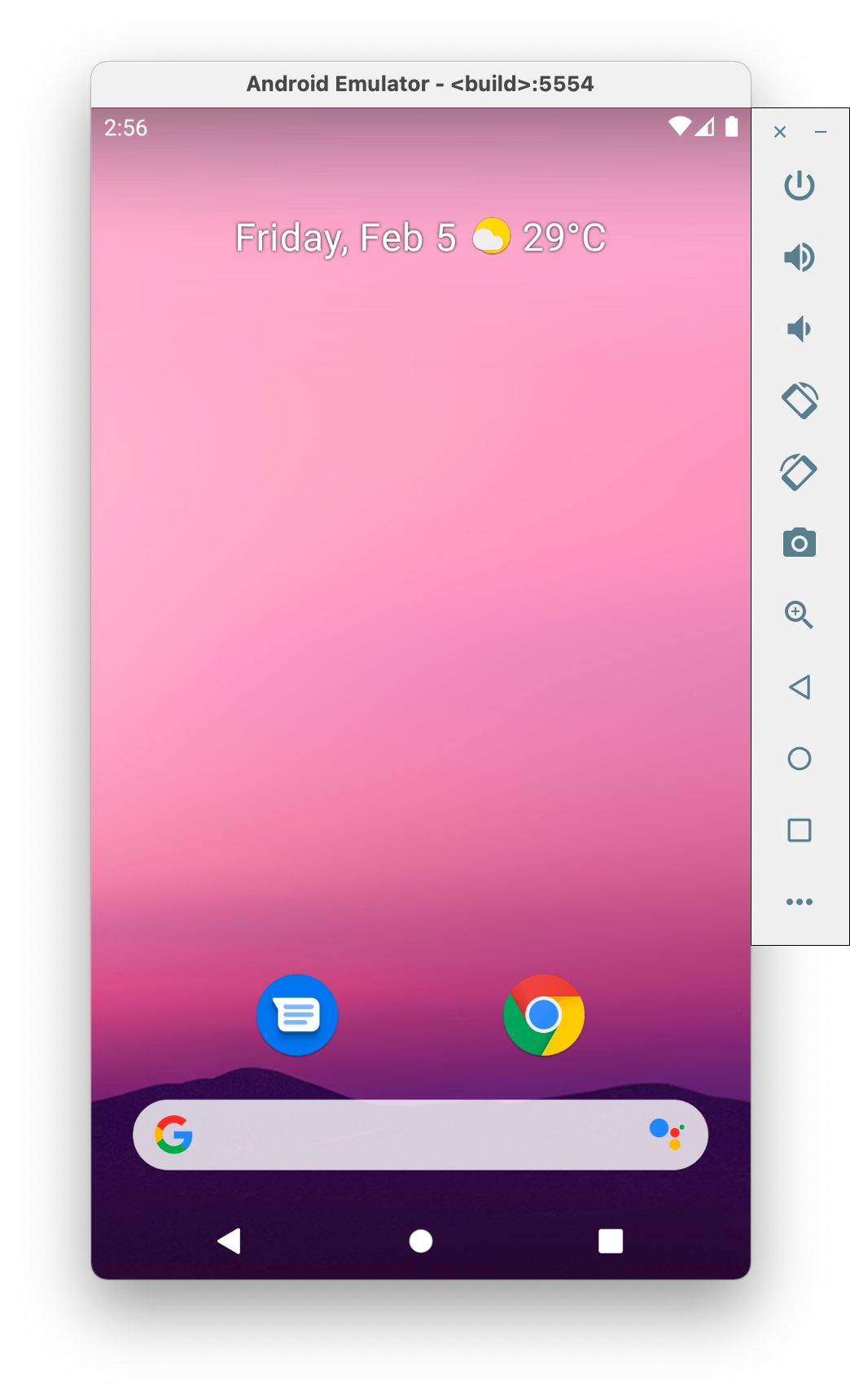The screenshot displays the home screen of an Android emulator, characterized by a serene gradient background that transitions from a pink sky at the top to deep purple hues and culminates in purple mountains at the bottom. At the very top of the screen, the time is prominently displayed as "2:56," accompanied by standard icons for reception and battery in the upper right corner. Below the time, the date reads "Friday, February 5th," alongside a weather update indicating "29 degrees Celsius" with an icon of a cloud partially obscuring the sun.

In the middle of the screen, there is a blue speech bubble icon, likely for a messaging or chatting application, situated next to the Chrome browser icon. At the bottom, a Google search bar spans the width of the screen, featuring the "G" logo on the left and the Google Assistant icon on the right.

The iconic Android navigation menu is positioned at the very bottom of the screen, comprising a left-facing white triangle (Back button), a white circle (Home button) in the center, and a white square (Recent apps button) on the right. Additionally, to the right of the main display, there is a docked control panel containing various utility buttons, including options for power, volume adjustment, screen tilting left or right, camera, magnifying glass (likely for search), a back button, and a vertical stack of the main navigation buttons, complemented by three dots at the very bottom for additional settings or options.